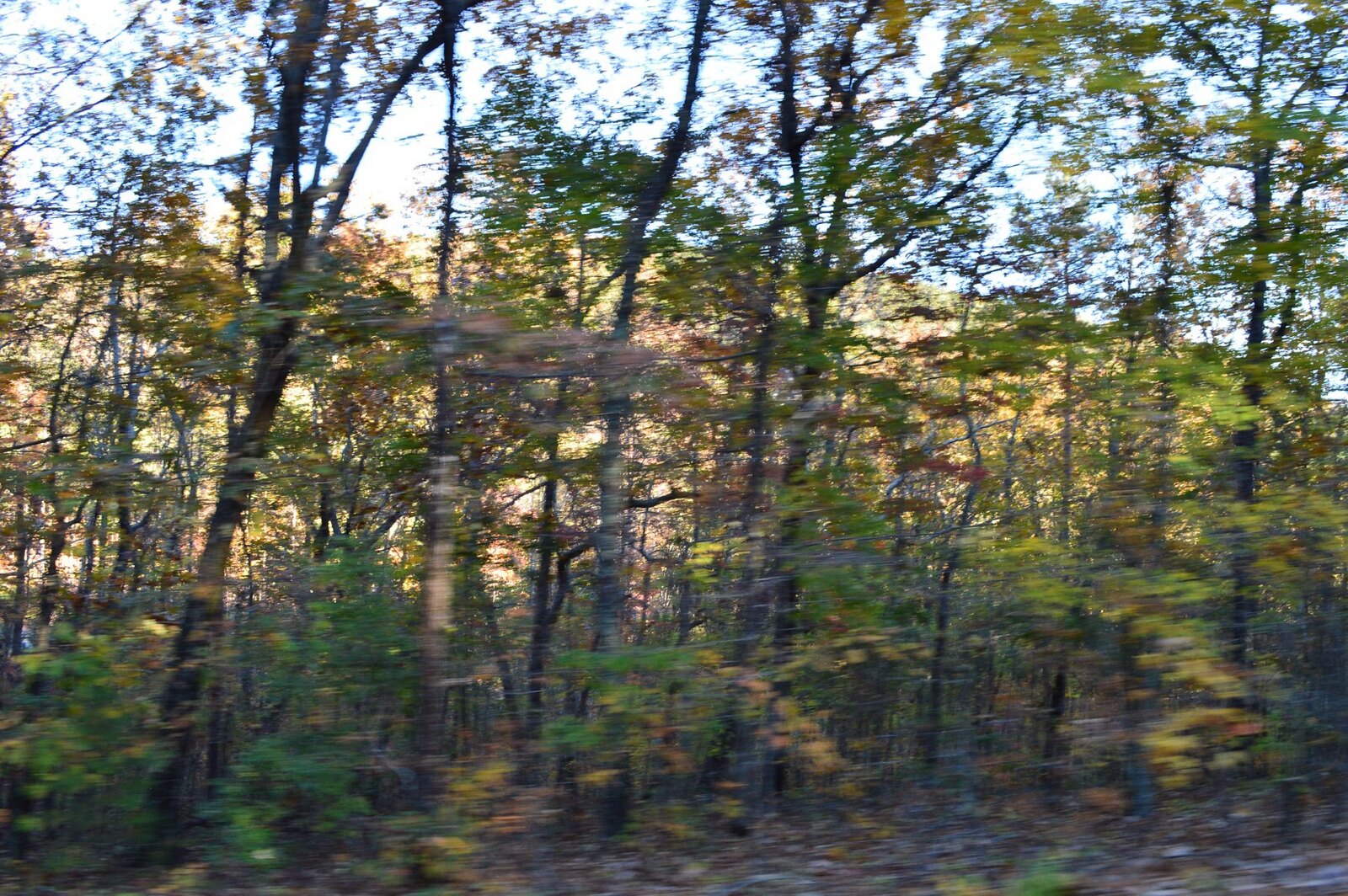An outdoor photograph captures a somewhat blurred scene of a lightly wooded forest in the early stages of fall. In the foreground, a variety of tall, thin trees with dark gray branches and a mix of green-yellow and brown leaves stand amidst a ground scattered with dead brown leaves. A particularly curved tree with a very dark trunk can be seen on the left. The canopy appears slightly thinning, indicating the onset of autumn. Through the trees, a low, slightly curved mountaintop bathed in sunlight is visible in the background, characterized by its bright yellow hue. The sky above is a light blue with a few clouds, partially visible through the treetops. The overall scene, depicting the changing colors of the season, is captured in daylight, giving the image a crisp yet slightly dreamy quality, suggesting it might have been taken from a moving vehicle.